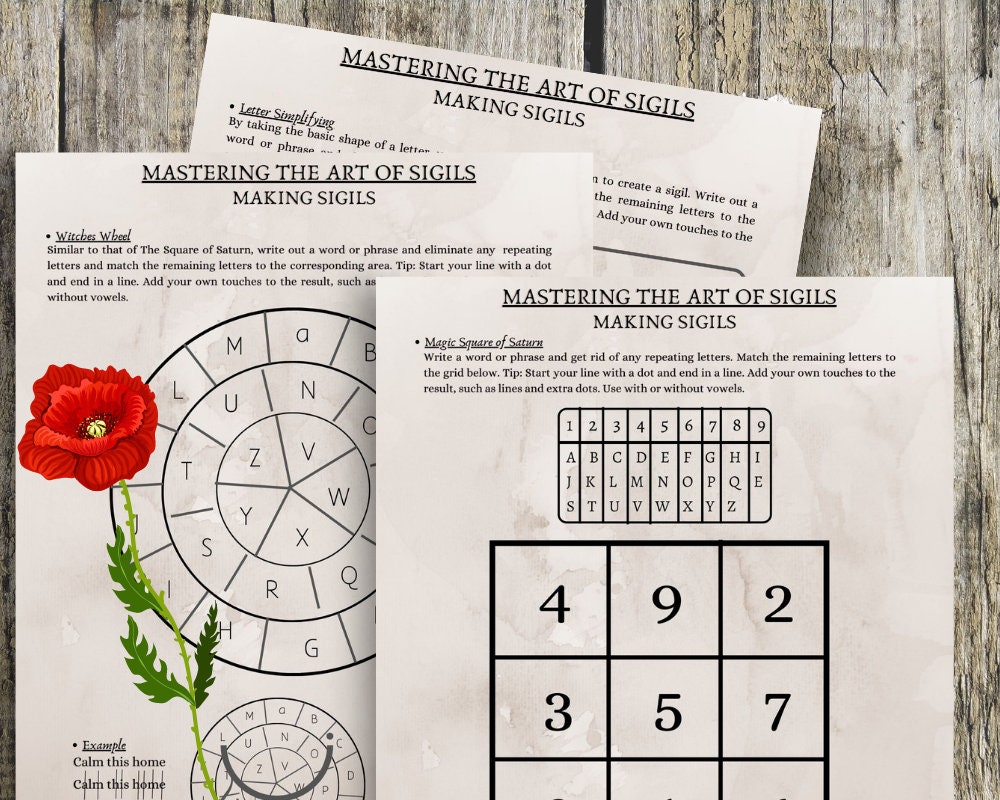The photograph captures three pages from a book titled "Mastering the Art of Sigils," each prominently labeled at the top. The pages lie on a wooden surface, possibly a table, with a slatted wooden fence in the background. Two of the pages overlap, partially obscuring the third. The visible headings include "The Magic Square of Saturn" and "Witch's Wheel," two prominent methods for creating sigils. The content of the pages consists of word and number puzzles that involve grids, charts, and key diagrams to aid in the completion of these mystical symbols. The top page features a colorful red rose with a green stem, contrasting strikingly with the otherwise black-and-white text and diagrams. The puzzles include detailed instructions on creating and solving sigils, such as letter simplification techniques and the usage of a circular diagram with concentric circles for generating codes or sigils. The overall layout suggests these might be assignments or exercises designed to practice the art of sigil-making.